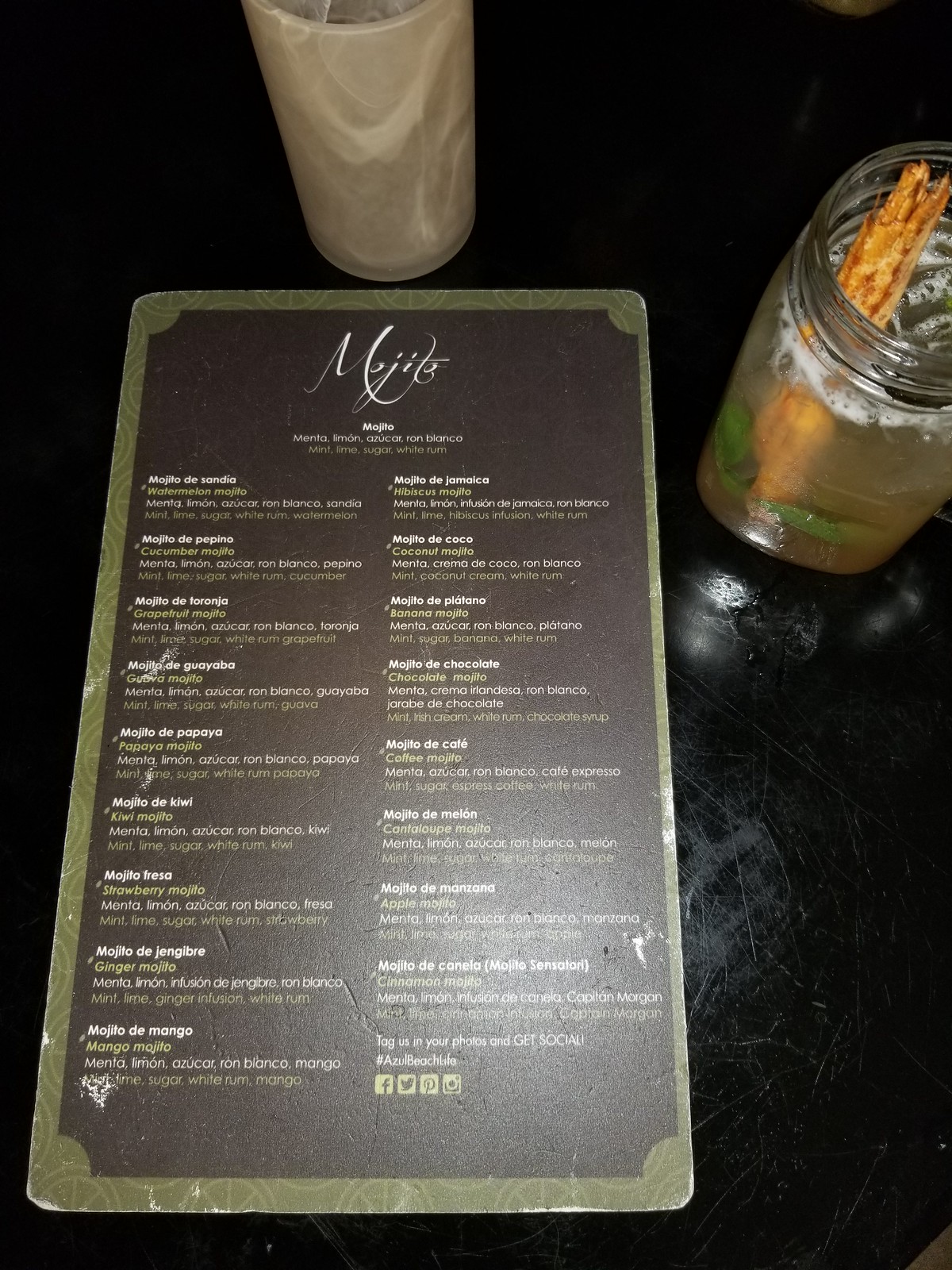A detailed menu and two beverages sit on a heavily scratched black table, which could be made of wood or metal. The lower right corner of the table is noticeably marred, while the upper edge appears smoother. The menu, positioned slightly left of center near the bottom edge of the table, features a gold trim and a brown background with elegant white font at the top, likely spelling out "menu" in either a stylized script or a foreign language. The menu layout displays two columns, each listing approximately nine items in white text.

Above the menu in the center of the image, the rounded base of a cup or glass can be seen, holding what seems to be a swirled white beverage. To the right, there's a clear mason jar filled with a brown liquid, possibly tea, adorned with cinnamon sticks and two green leaves resting at the bottom left inside the jar.